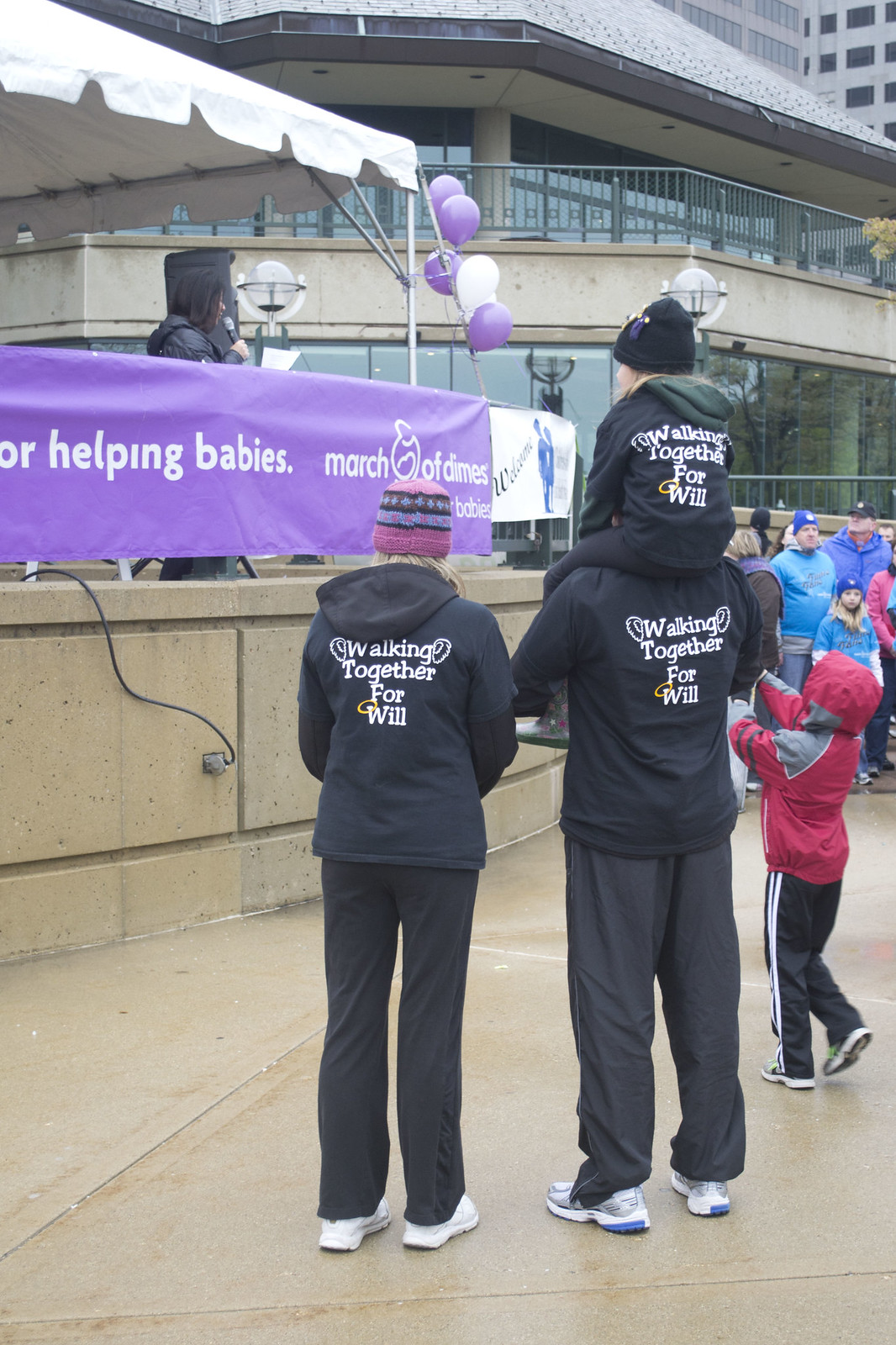The image captures an outdoor rally with a speaker standing on an elevated platform under a portable tent, holding a microphone and addressing the crowd. The speaker is positioned to the left, wearing a black coat with the hood up. A large purple banner in front of the speaker reads, "Helping Babies, March of Dimes," accompanied by an array of purple and white balloons attached to the canopy. In the foreground, a family of four takes center stage, all donning matching black t-shirts that read "Walking Together for Will." The mother, identifiable by her pink patterned beanie and blonde hair, stands to the left, while the father, wearing gray joggers and white trainers, stands to the right with their son on his shoulders, also wearing the same t-shirt. A small girl with a black beanie and a boy in a red and gray coat also appear in the scene. The family and scattered children face the speaker, set against the backdrop of tall buildings. It’s a lively scene brimming with community spirit and a shared purpose to support the cause.